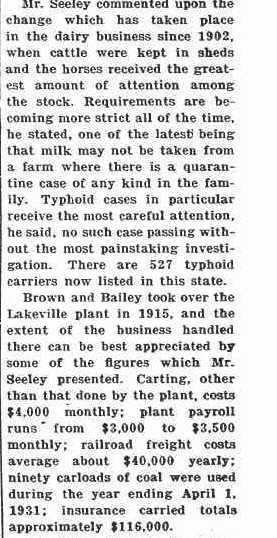This image is a close-up photograph of an old newspaper article featuring black text on a white background. The article is displayed in a single column justified to both the right and left. A thin black line runs vertically along the left side, partially cutting off the text. The article consists of two paragraphs.

The first paragraph reads: "Mr. Seeley commented upon the change which has taken place in the dairy business since 1902, when cattle were kept in sheds and the horses received the greatest amount of attention among the stock. Requirements are becoming more strict all the time, he stated, one of the latest being that milk may not be taken from a farm where there is a quarantine case of any kind in the family. Typhoid cases, in particular, receive the most careful attention, he said, no such case passing without the most painstaking investigation. There are 527 typhoid carriers now listed in this state."

The second paragraph details the business operations of the Lakeville plant: "Brown and Bailey took over the Lakeville plant in 1915 and the extent of the business handled there can be best appreciated by some of the figures which Mr. Seeley presented. Carting other than that done by the plant costs $4,000 monthly; the plant payroll runs from $3,000 to $3,500 monthly; railroad freight costs average about $40,000 yearly. Ninety carloads of coal were used during the year ending April 1, 1931, and insurance carried totals approximately $116,000."

Overall, the image presents a historical account of changes in the dairy business and operational specifics of the Lakeville plant, richly detailed with financial figures and regulatory updates from the early 20th century.